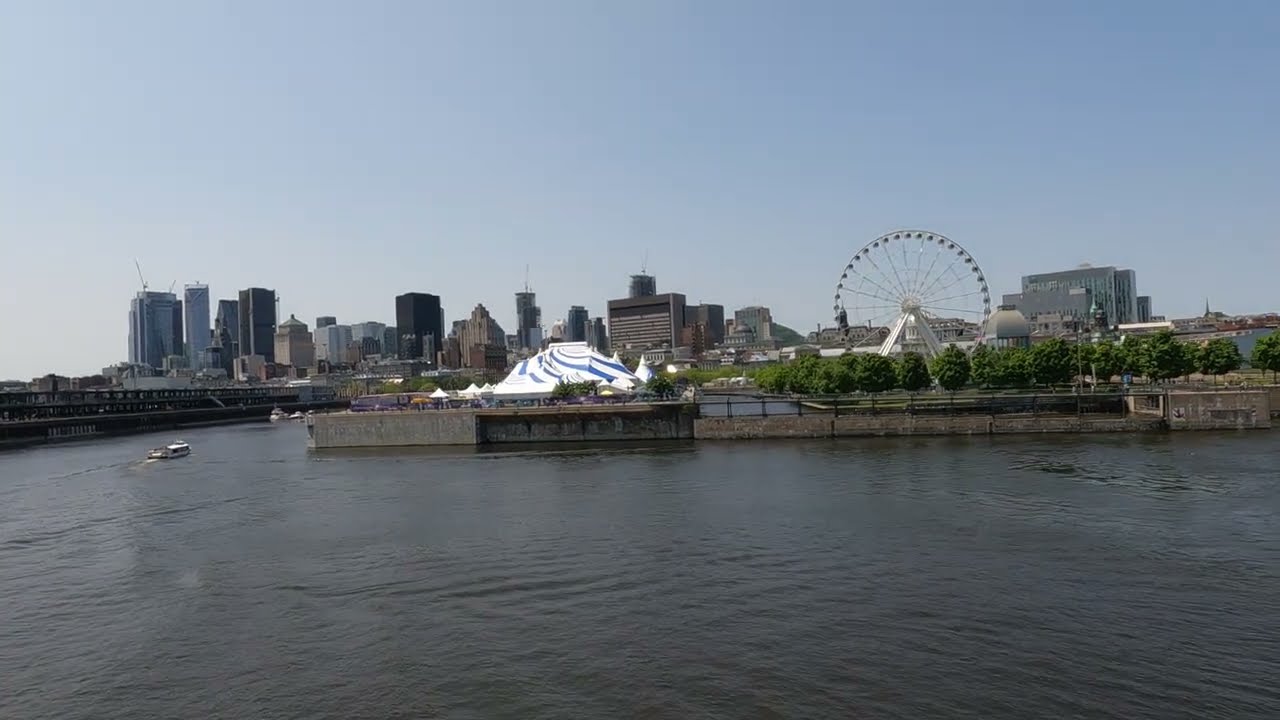The photograph captures a lakeside cityscape on a somewhat hazy, sunny day. In the foreground, dark, slightly wavy water extends towards a concrete pier-like shoreline, which is furnished with chairs and tables under a white tent. To the left side of the image, a small boat with a covered area, possibly for tourists, gently rests on the water. The city skyline stretches across the middle of the image, featuring an array of tall buildings, none distinctly taller than the others. Off to the right, a large ferris wheel commands attention as a central focal point. The sky above is a hazy shade of blue, adding a muted, serene backdrop to the bustling city panorama below. The primary colors in the scene are shades of blue, gray, white, and a hint of green from the water, giving it a tranquil yet vibrant ambiance.